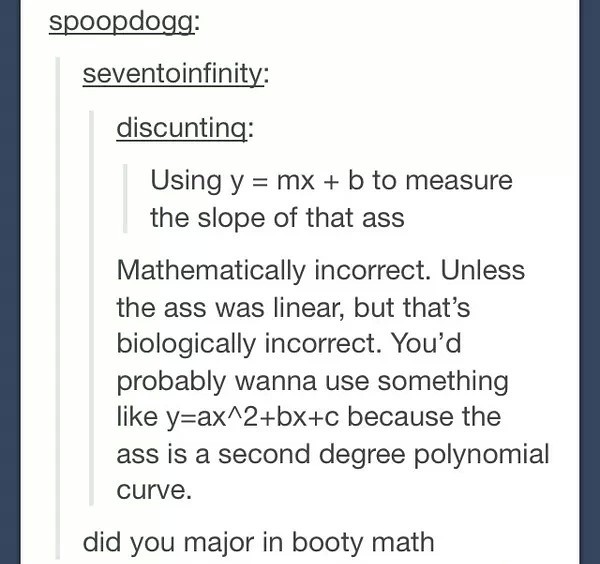The image is a screenshot of a social media post, possibly from Reddit or Tumblr, featuring humorous comments discussing the mathematical representation of a curve. At the top of the post, there is a header with the username "Spoopdog" followed by "7 to infinity" and what seems to be the word "discounting." The primary comment humorously suggests using the linear equation \( y = mx + b \) to measure "the slope of that ass." A reply corrects this by noting that such a linear equation is mathematically and biologically incorrect for describing a natural curve, proposing instead the quadratic equation \( y = ax^2 + bx + c \) as a more accurate model for a second-degree polynomial curve. A third person joins the thread with a witty remark, "Did you major in booty math?" The background remains plain white with simple black lettering, giving the humorous mathematical exchange a clean, minimalistic appearance.